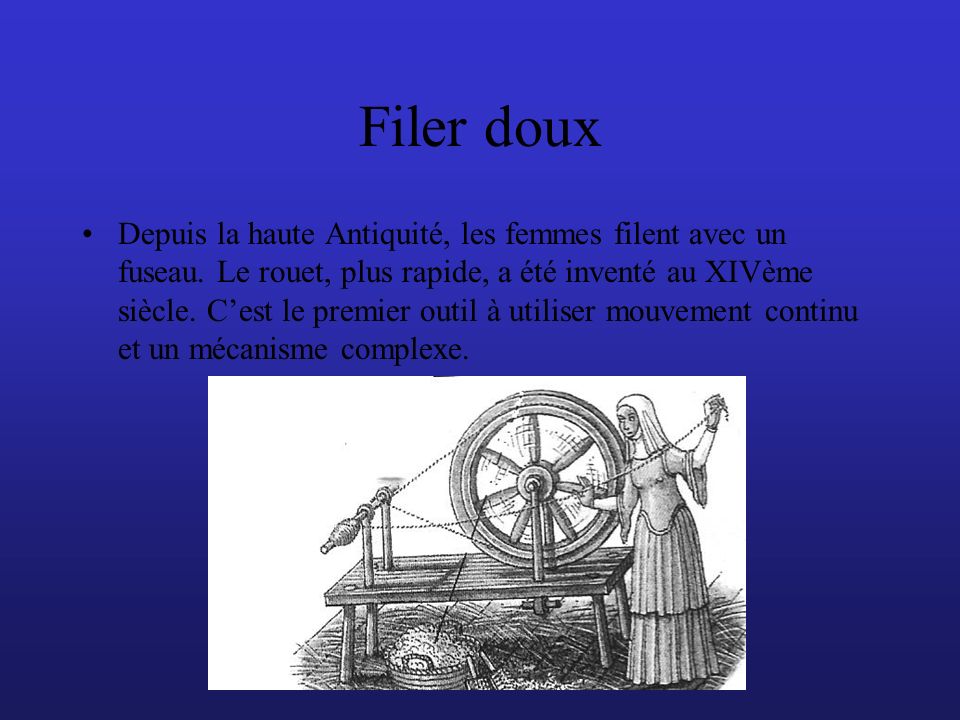The image depicts a presentation slide with a blue gradient background, becoming darker from top to bottom, reminiscent of a PowerPoint design. At the top, in black text, it reads "Filer d'eau", followed by a bullet point and a lengthy paragraph in French. The text translates to a historical context about women using a spindle since ancient times. Below this text is a detailed black and white illustration of a medieval woman. She wears a headscarf and a long dress, working at a large wooden sewing wheel. The scene includes a wooden table, a basket of yarn to the left, and a floor with scattered straw, emphasizing the antiquated setting. The woman, resembling a nun, operates the spindle, threading fabric through it, demonstrating an old textile fabrication process.